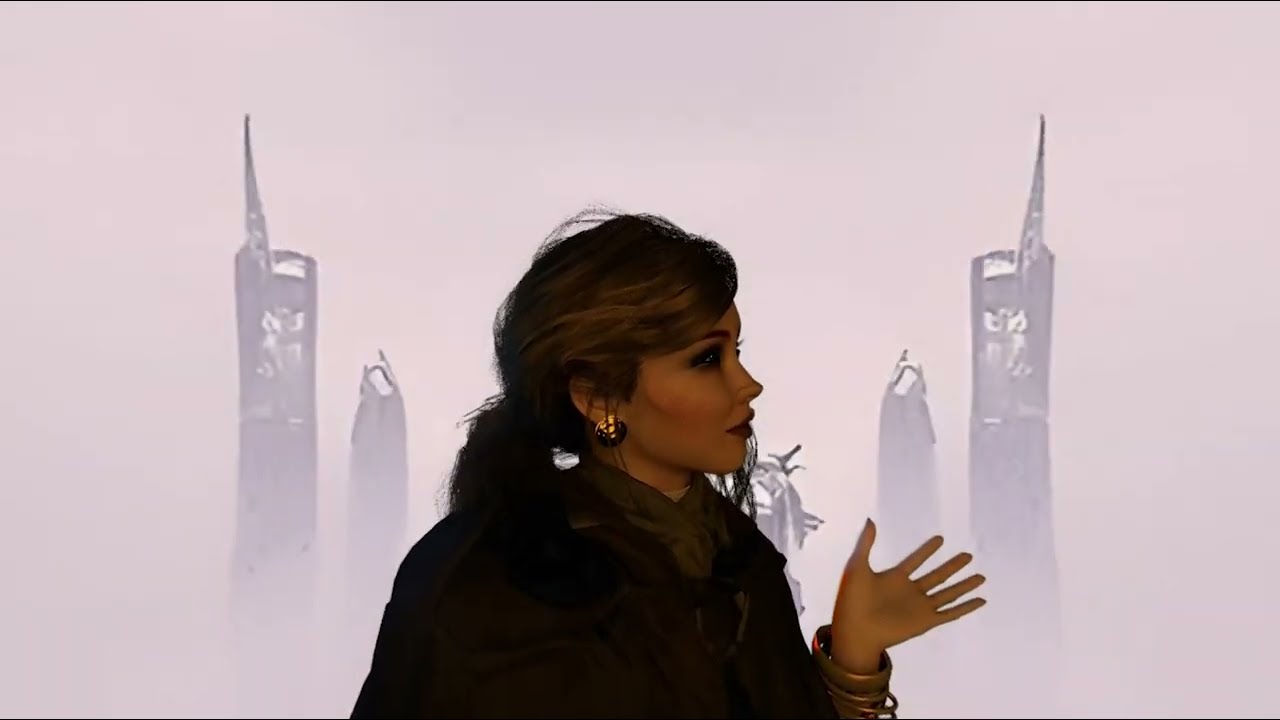In the image, a young woman stands prominently in the center, facing sideways to the right. She has long, dark brown hair tied in a low ponytail and wears gold bracelets on her left hand, which is open and facing upwards. She is dressed in a dark shirt with a jacket or blouse over it. Her appearance is complemented by gold-colored earrings and dark lipstick. The background features a foggy, computer-generated cityscape with several diffused, overcast skyscrapers, creating a smoky and light pink to gray ambiance. The setting appears to be part of an indoor presentation or video game scene, characterized by a tannish, smoky, and abstract design without any discernible text.